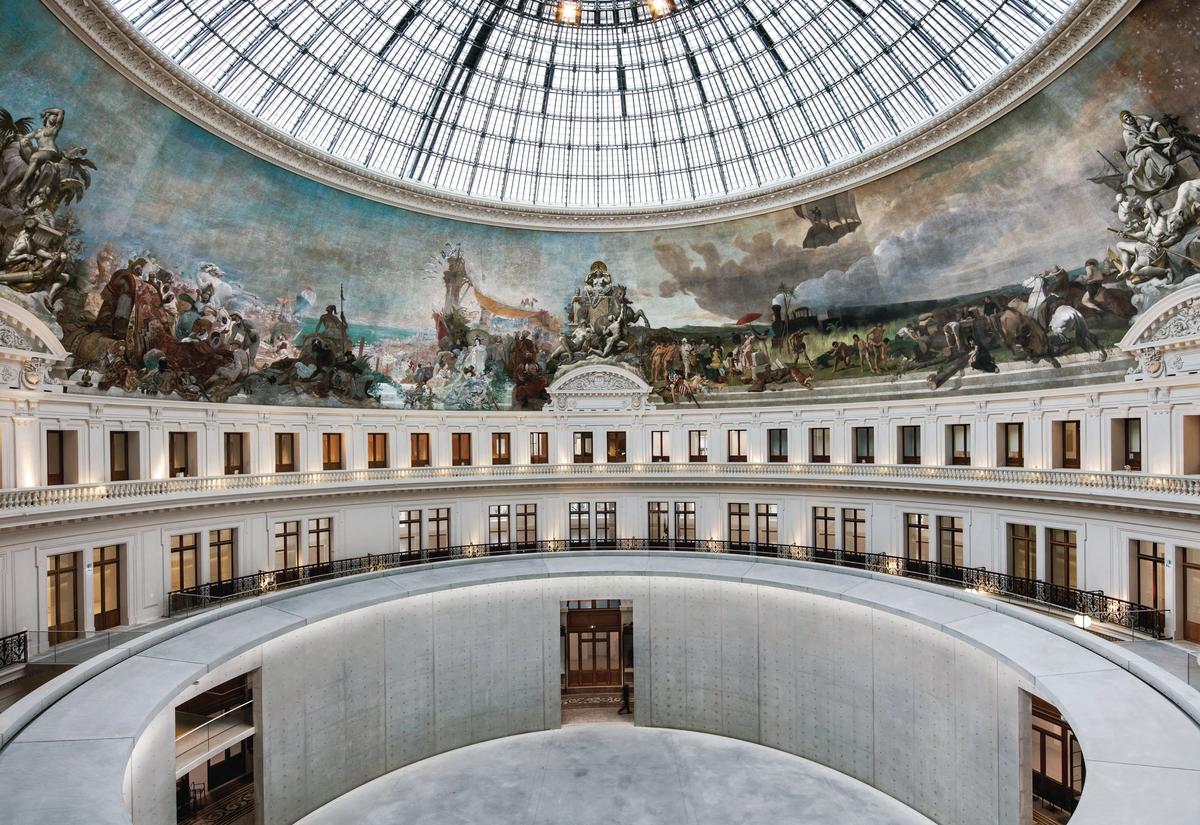In an expansive and grandiose rotunda, likely part of a government or state Capitol building, the scene reveals a quiet, possibly after-hours interior with no people present. The entire space showcases impressive architectural detailing and artistry. The floor is made of polished marble, creating a circular layout that directs attention upwards. Encircling the room on the second floor are numerous windows, repeating around 10 to 12 times, which illuminate the space with natural light that filters through the glass dome at the very top. Above the second floor, a third-floor railing suggests an additional tier, albeit likely narrow, further enhancing the verticality of the structure. Covering the uppermost section of the rotunda is a vast fresco featuring dynamic scenes of soldiers or people in combat, some on horseback, which adds a vibrant historical or mythical narrative to the space. The fresco weaves around the dome just below the glass apex, allowing light to flood the intricate artwork. The overall ambiance is one of solemn grandeur, steeped in history and significance, with architectural and artistic details meticulously interwoven throughout the rotunda.